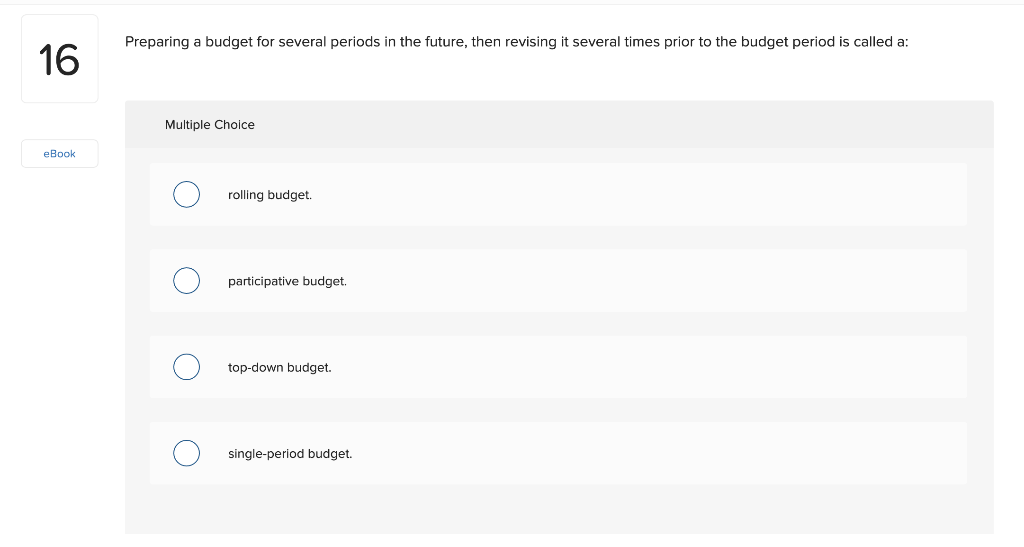This screenshot captures a section of a questionnaire displayed against a crisp white background. At the top, a thin horizontal light gray line spans the width of the image. Just below and to the left, a white square with a thin light gray outline and rounded corners prominently features the large black number "16". Directly beneath this is a shorter white rectangle, also with a thin light gray outline and rounded corners, containing blue text that reads "e-book" with an uppercase "B" and the rest of the letters in lowercase.

To the right of the number "16", a line of small black text reads: "Preparing a budget for several periods in the future, then revising it several times prior to the budget period is called:" followed by a colon. 

A couple of line breaks down, the image reveals a large light gray rectangle. This rectangle includes a slightly darker gray header at its top left corner, where small black text reads: "multiple choice". Directly below within the light gray rectangle, there are four even lighter gray rectangles, each separated by small areas of negative space. Each rectangle features a white circle with a thin dark blue outline on its left side. To the right of each circle, small black text delineates the multiple-choice options, ending with a period. From top to bottom, these options read: "rolling budget.", "participative budget.", "top-down budget.", "single-period budget.". The overall layout is clean and organized, ensuring each element is clearly separated by negative space.